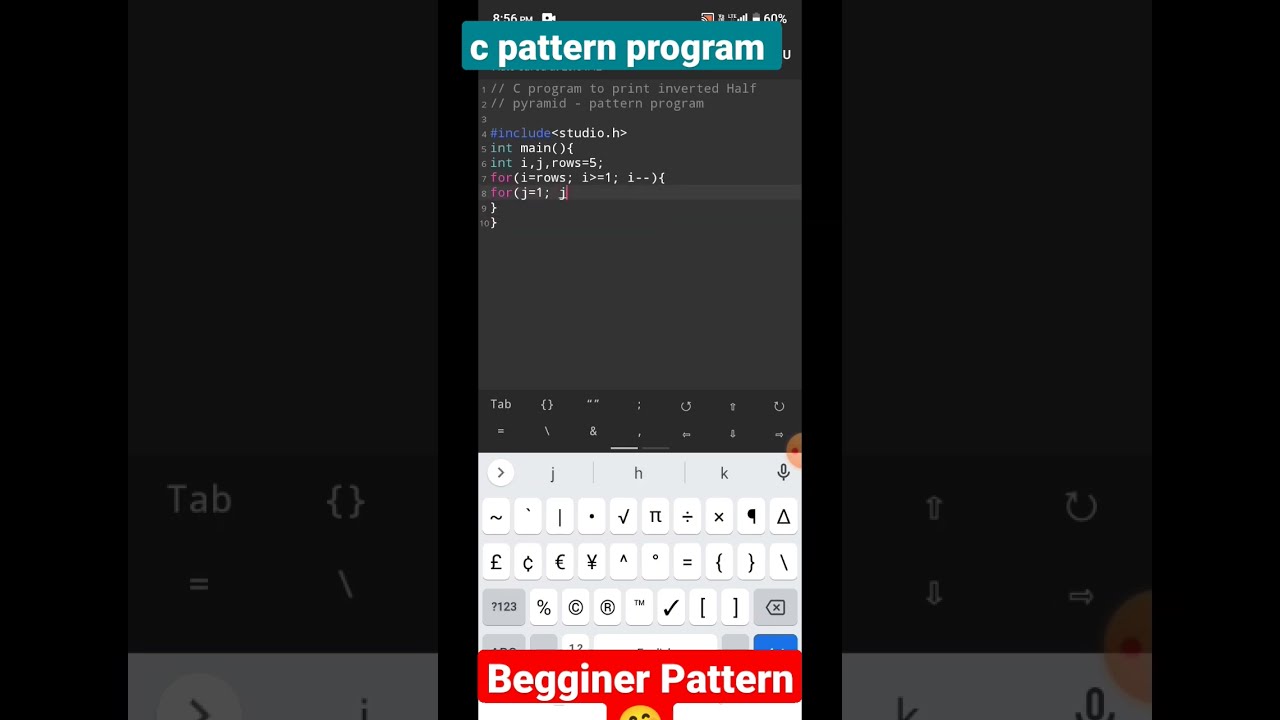The image is a composite made up of three distinct rectangles. The central vertical rectangle is the primary focus, showcasing a smartphone screenshot. At the very top of this section, a turquoise tab with white lettering reads "C-Pattern Program." Below this is a black screen filled with lines of computer code featuring a variety of colors: gray, blue, green, and purple. Additional details at the top of the screen display the time, battery percentage, and signal strength typical of a smartphone interface. Following the code portion, there's an overlay of a keyboard with special icons activated, including a glimpse of a smiley emoji at the bottom. A red horizontal rectangle with white text saying "Beginner Pattern" overlays the keyboard section. The image appears to have been enlarged and darkened, with the left and right edges displaying the black portions of the originally larger background showing some tab labels and special function keys.